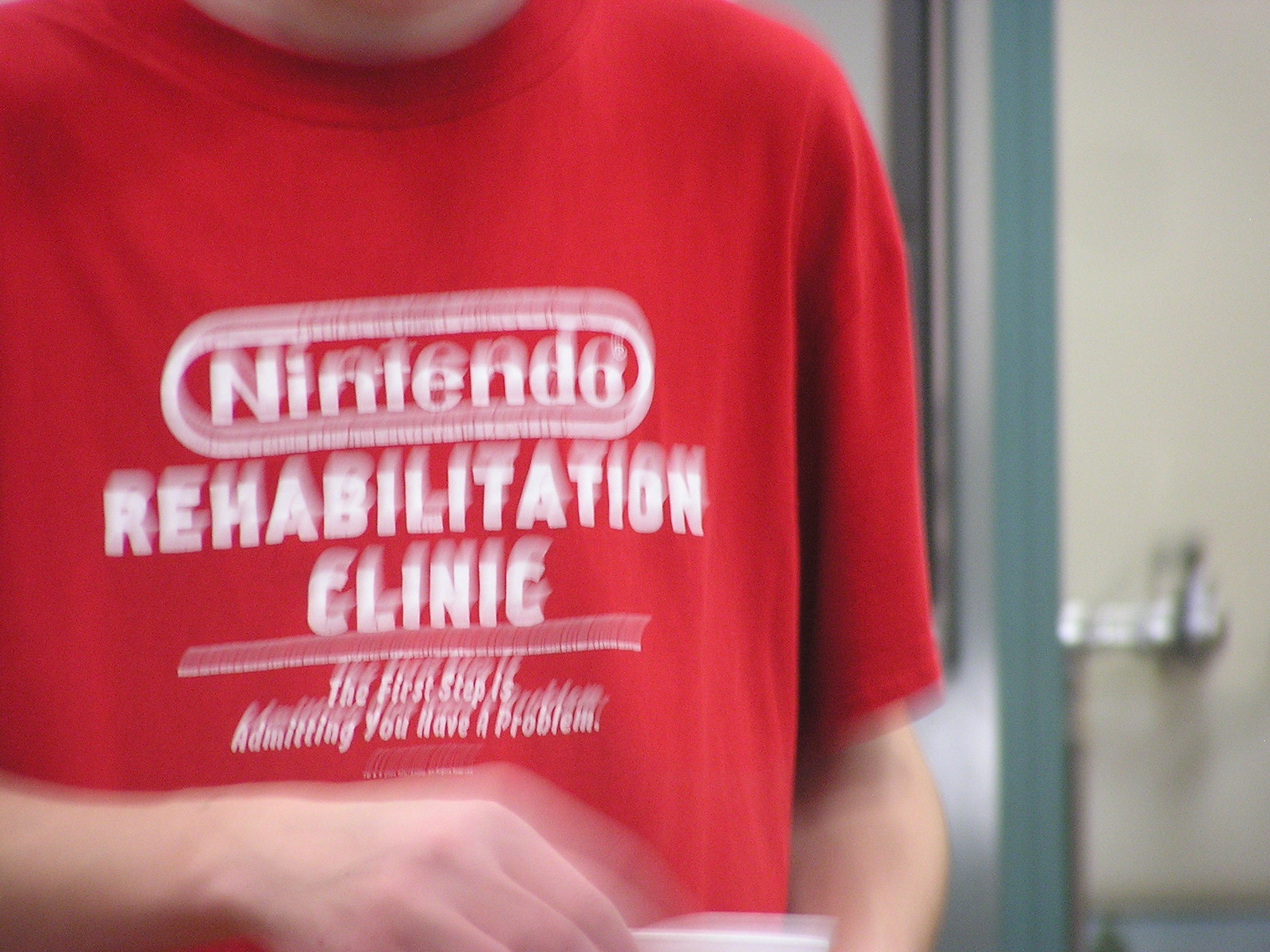A blurred photograph captures the upper torso and right hand of an individual. They are dressed in a red shirt adorned with white lettering that prominently displays the Nintendo logo at the top. Below the logo, the shirt reads, "Rehabilitation Clinic," and further down, it states, "The first step is admitting you have a problem." The person's left elbow is also visible in the frame. They seem to be holding an indistinguishable object in their right hand. The background features an ivory-colored door with green trim and a silver doorknob.